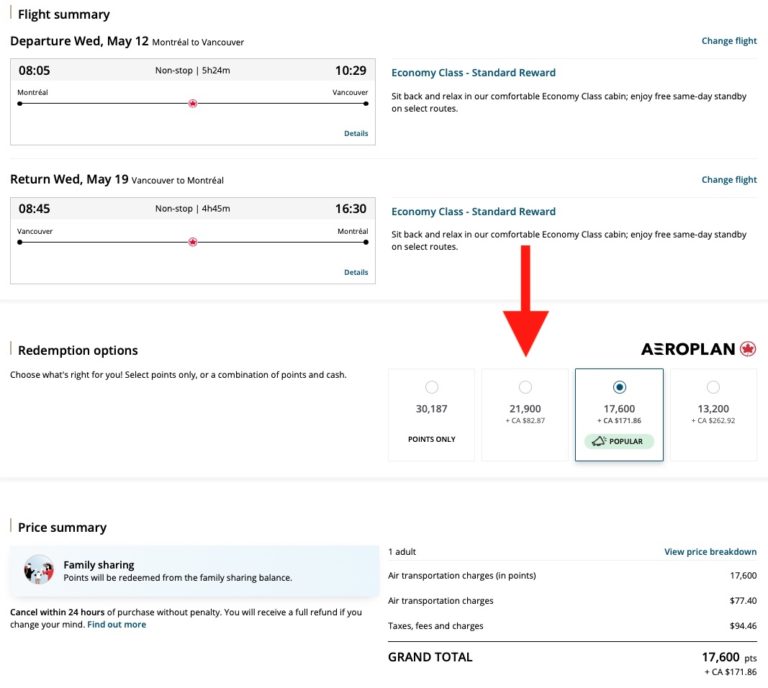The image captures a detailed flight booking summary on an airline website. At the very top left, "Flight Summary" is prominently displayed in black text. Directly below, the departure information is listed: "Wednesday, May 12th, Montreal to Vancouver." This section includes a detailed rectangular box indicating flight timings and durations. 

The top left of this box displays "08:05" while the top right shows "10:29." Centrally aligned at the top is a label stating: "Non-stop, 5 hours and 24 minutes." Under the time "08:05," the text "Montreal" is accompanied by a small black circle, with a line extending to "Vancouver" on the right. The bottom right corner of this box contains a "Details" link.

Below this, the return flight details are presented: "Wednesday, May 19th, Vancouver to Montreal." This section mirrors the departure details with timings "08:45" to "16:30" and a note indicating the same non-stop duration format.

On the bottom left of the image, a section titled "Price Summary" is visible. Within a blue-hued box, "Family Sharing" is mentioned, noting that "Points will be redeemed from the Family Sharing balance." The bottom right corner houses the financial details, specifying the grand total as "917,600 points."